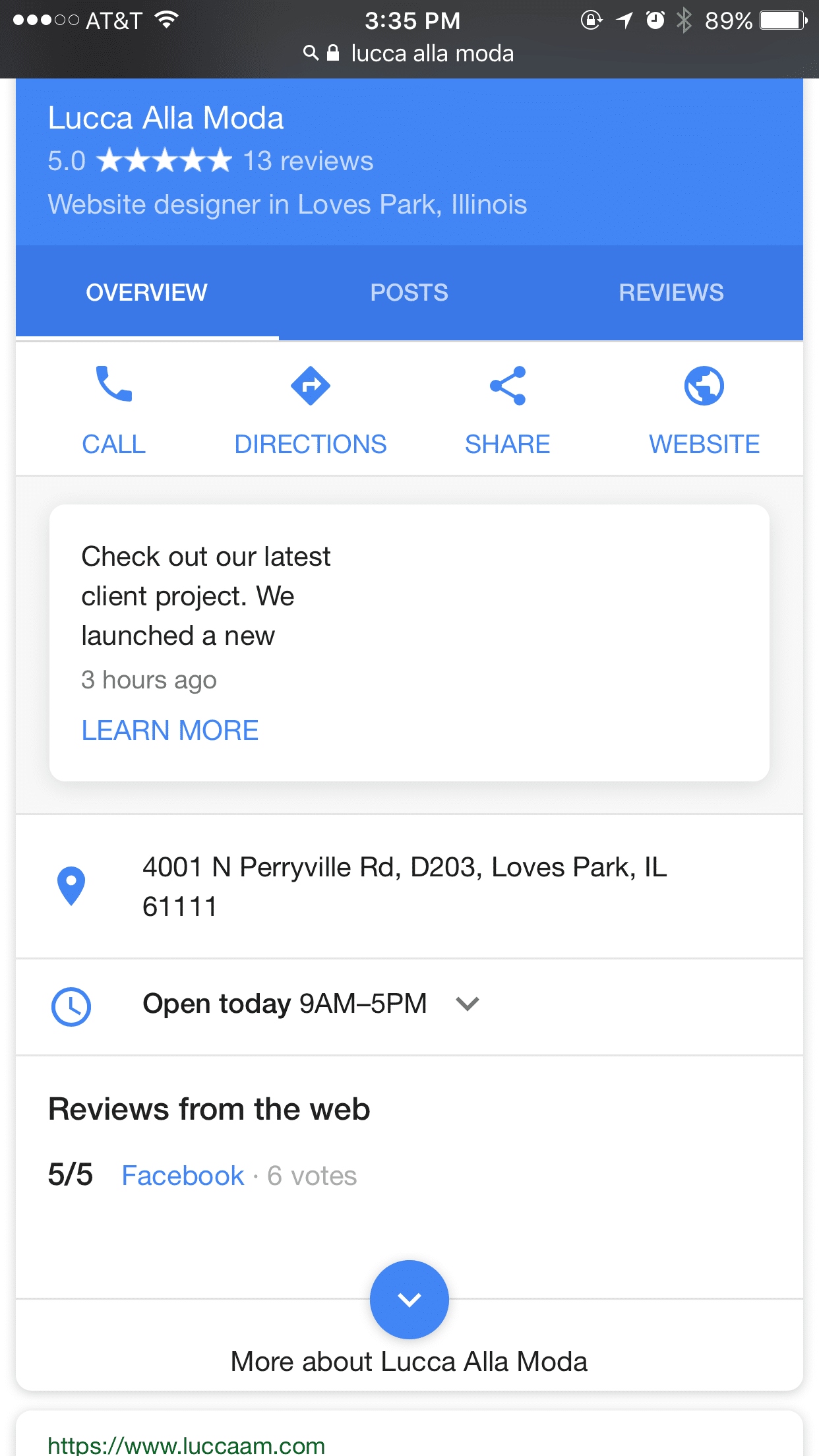The image features a light blue background with a black bar at the top, displaying three filled-in white circles, indicating signal strength, AT&T as the network provider, the time of 3:35 PM, and an 89% battery level. Below this, there is a prominent blue box showcasing "Luca a la mode" with a five-star rating. It identifies Luca a la mode as a website designer based in Loves Park, Illinois. Navigation options such as "Overview," "Posts," and "Reviews" are visible.

Additional blue buttons in the lighter blue section offer options for "Call," "Directions," "Share," and "Website." A featured announcement highlights the launch of a new client project three hours ago, with a prompt to "Learn More." The company’s address, "4001 North Cherry Hill Road, D203, Loves Park, Illinois, 61111," is listed along with business hours of "Open today 9 to 5." Web reviews praise Luca a la mode, giving it a strong 5 out of 5 rating. A blue circle with a down arrow invites users to learn "More about Luca a la mode," and the URL "http://www.luca.com" is provided for direct access to their website.